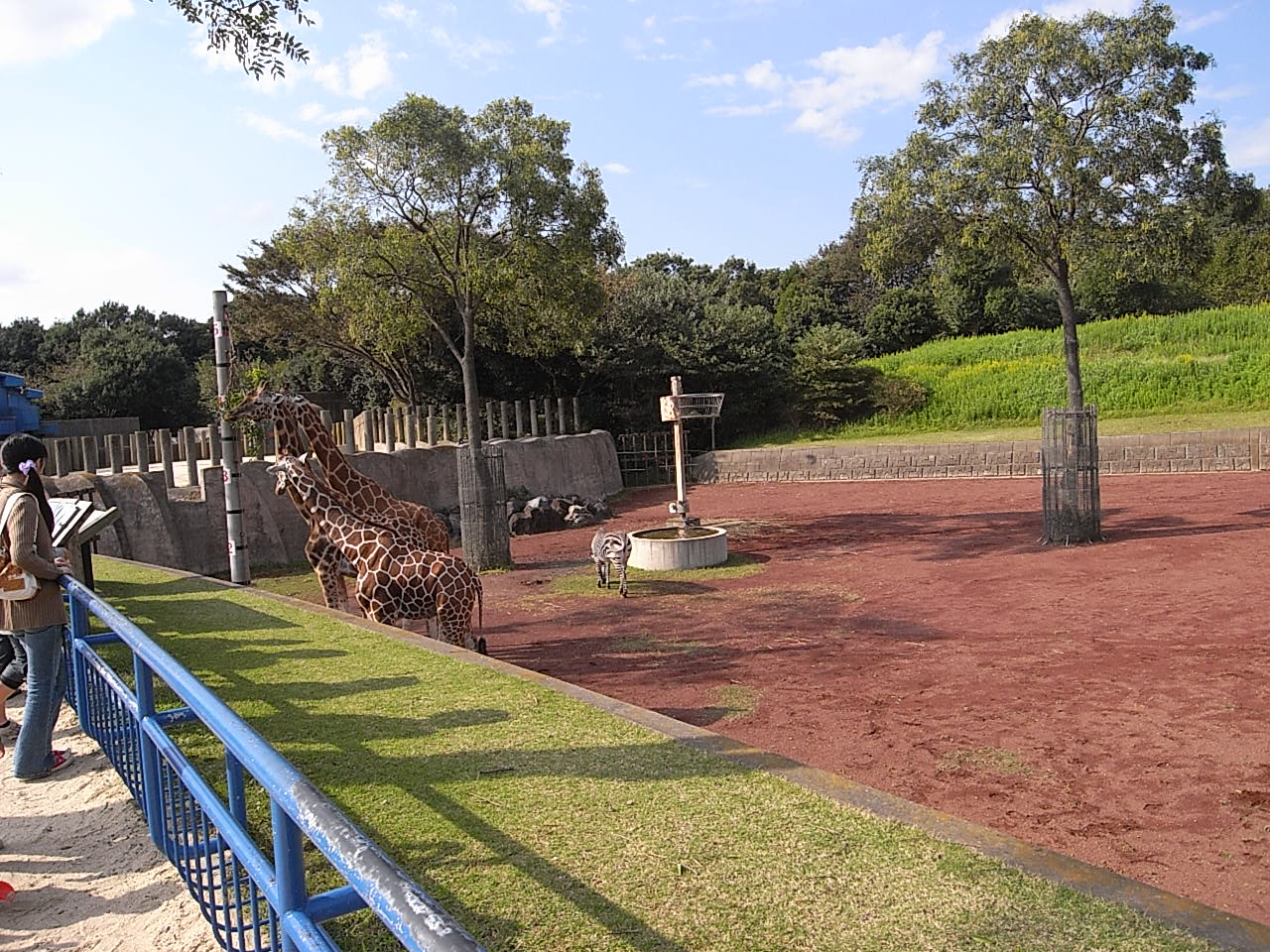The photograph captures a vibrant, sunny day at a zoo from the perspective of a visitor. In the foreground, there's a blue steel railing with a woman in jeans and a jacket standing against it, her black hair tied in a low side ponytail. She appears in profile view, partially cut off on the left edge of the image. Behind the railing, several visitors are lined up, their shadows cast heavily on the green grass due to the bright sunlight.

Beyond the railing lies an open animal enclosure that emulates a savannah, bordered by a green embankment and dropping into a pit of red clay dirt. The enclosure features two or three giraffes, some of which are eating leaves from a tall, gray feeding pole, and a single zebra grazing on a small patch of grass next to a large white concrete water trough. The area is dotted with a few trees protected by small fences, adding to the simulated natural habitat. The background shows more greenery, walls, and possibly a berm with additional trees and bushes. The bright blue sky, speckled with a few white clouds, completes this picturesque scene at the zoo.